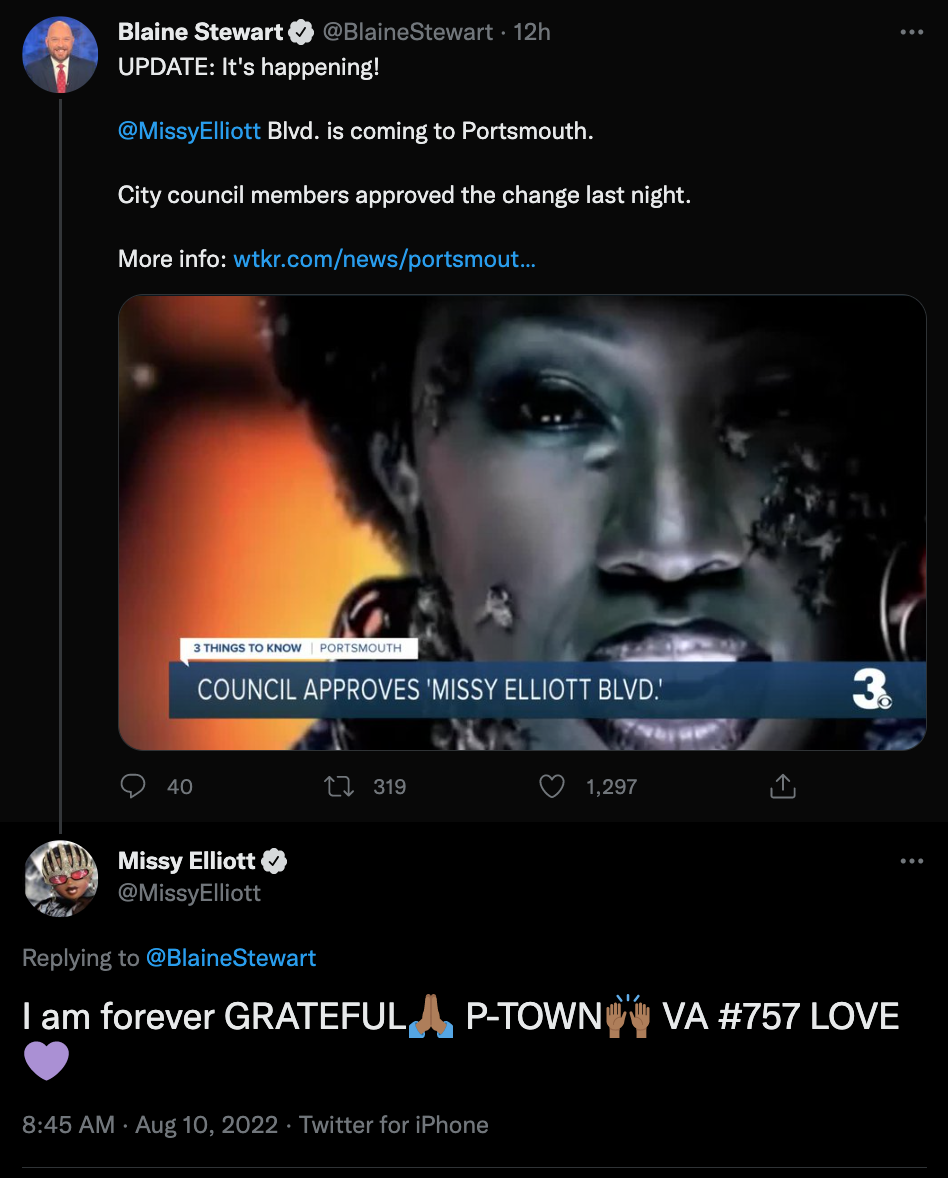A Twitter screenshot displays a post from Blaine Stewart, who is verified with a checkmark next to his name. His profile picture shows him in a suit. The post, made 12 hours ago, features the following text: 

"Update: It’s happening. Missy Elliott Boulevard is coming to Portsmouth. City council members approved the change last night. More info: [WKTR Link]"

Below this text, there is a screenshot of Missy Elliott with gray face paint. Accompanying this image is a news headline that reads, "Council approved Missy Elliott Boulevard." Underneath the headline, Missy Elliott's comment from her Twitter account is shown, stating, "I am forever grateful P-Town VA #757 love."

[Image description: Blaine Stewart's tweet and explained news screenshot featuring Missy Elliott]